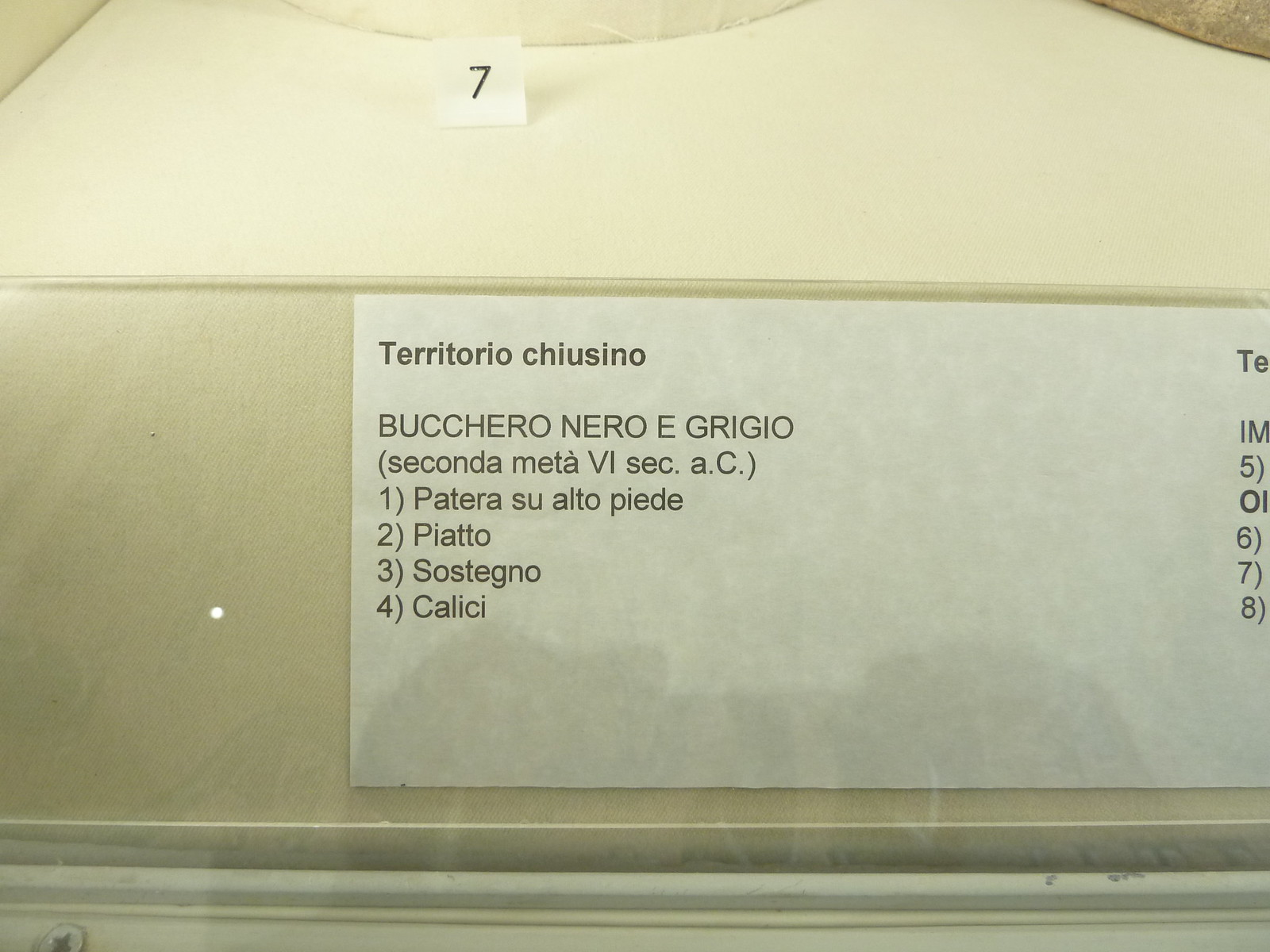The image features a zoomed-in view of a glass-encased display, likely set indoors, possibly within a restaurant or another building. The display contains a sign centrally positioned against a white background. The sign, written in a non-English language, reads "Territorio Chiusino" at the top, followed by "Bucero Nero e Grigio," with "Secunda Metavisec AC" in parentheses beneath it. Further below, a list enumerates items: "1. Patera Sueltapied," "2. Piatto," "3. Sostegno," and "4. Calice." Another card positioned at the top of the display bears the number seven, with a small semicircle above this number and a partially visible semicircle to the right. The background includes a wooden ledge at the bottom, secured with a visible screw in the lower-left corner. The colors in the image consist primarily of shades of brown, white, off-white, and black.